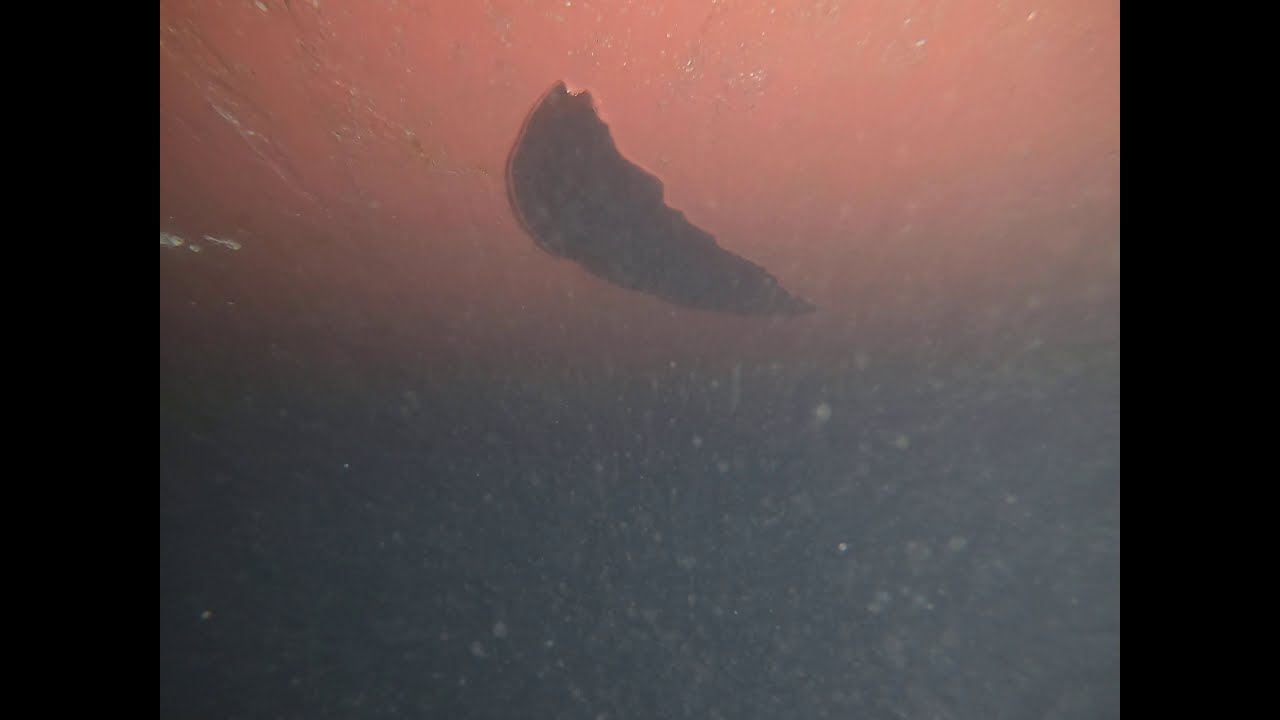The image is a hazy, out-of-focus photograph that seems to be taken through an unclear, dusty, or scratched medium, possibly a window. The picture is characterized by a gradient of colors, transitioning from a reddish, coral, sunset-like hue at the top to a nearly black, dark gray at the bottom. This gradient gives the appearance of a sunset or an underwater scene. The top section of the image, which exhibits a pinkish hue, houses an irregular, broken crescent-shaped object, dark in color, with a rounded edge on one side and a jagged, broken edge on the other. The entire image is covered in white specks and blotches, reinforcing the dirty, opaque quality. The overall impression is of a very blurry and dirty image, with poor lighting and indistinguishable details, making it difficult to determine the exact nature of the objects or scene depicted.